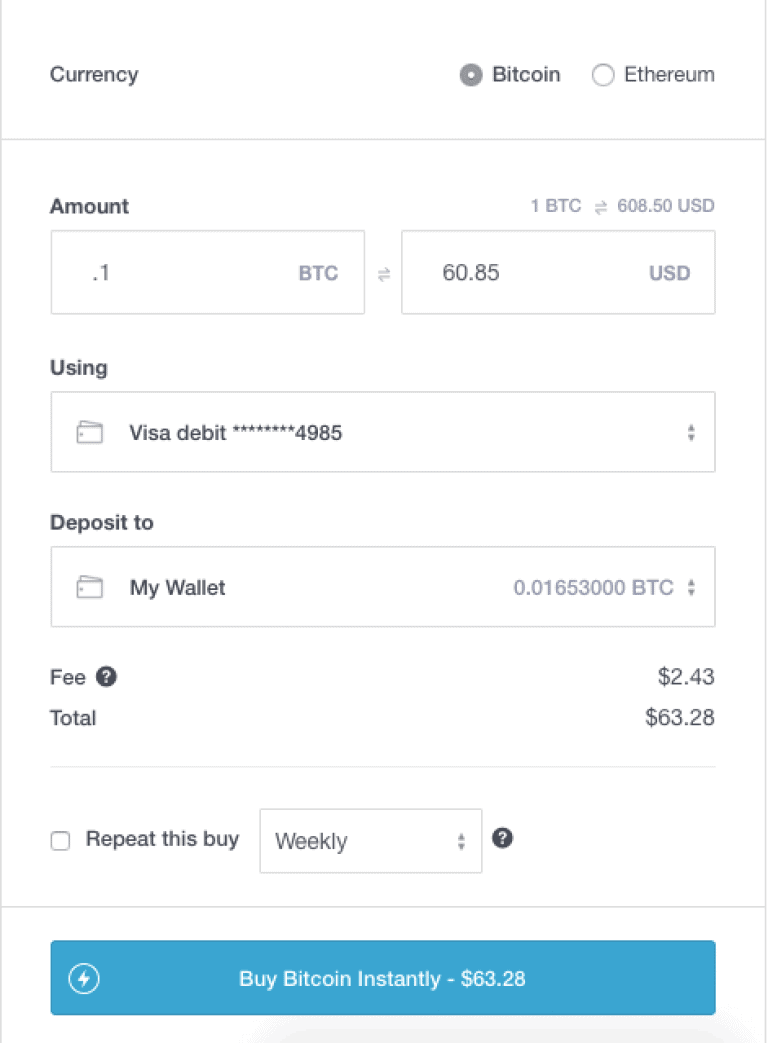This image appears to be a screenshot from a cryptocurrency exchange website. The interface predominantly features black text on a white background. At the top left corner, there are options to select between different cryptocurrencies, with Bitcoin already chosen and Ethereum available to the right.

Below this section, there's a field indicating the amount of Bitcoin to be transacted, showing an example value of 0.1 BTC, which corresponds to 60.85 USD. Above this, the current exchange rate is displayed as 1 BTC equalling 808.50 USD.

Further down, there is another field which seems to be for inputting or selecting a payment method, exemplified by "Visa debit ...4985" from a drop-down menu. The transaction is being deposited into the user's wallet, displaying a deposit amount of 0.01653000 BTC.

Additional information includes a fee, highlighted by a question mark icon for further details, noted as 243. The total for this transaction is listed as 6328 dollars. There is a checkbox option at the bottom allowing the user to repeat the transaction bi-weekly.

At the very bottom, a prominent rectangular button with 'Buy Bitcoin Instantly' and the amount $6328 in white text is displayed. To the left of this button, there is a small circle with an upward arrow, suggesting a functionality related to confirming or submitting the transaction.

Overall, this page is part of a financial or banking platform dedicated to Bitcoin transactions, facilitating the purchase and deposit of Bitcoin into the user's wallet.